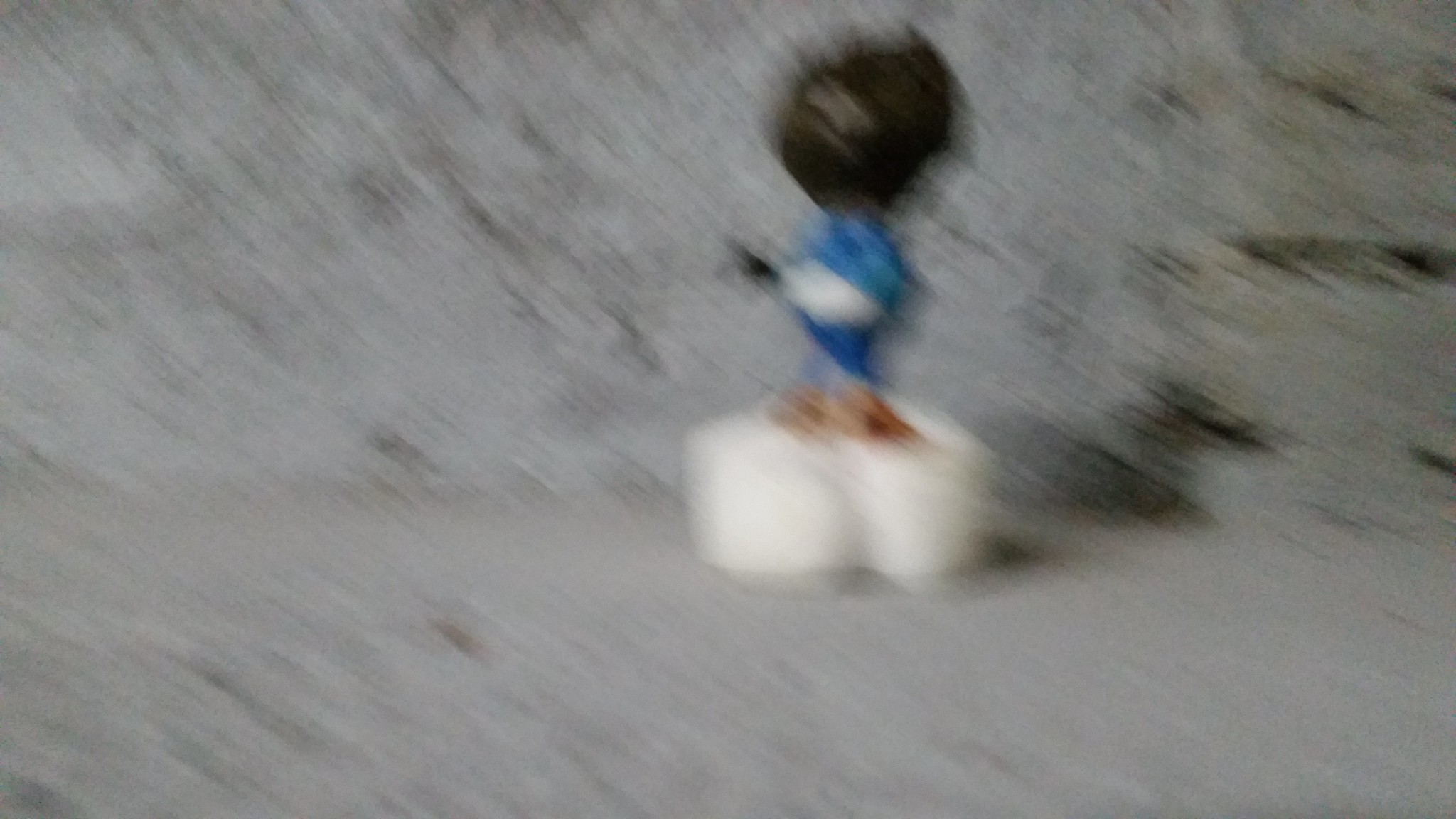The image depicts a very blurry figure standing against a grayish background with various darker gray splotches, suggesting a cement floor. The figure appears to be a small toy or figurine placed on something white, which might have the shape of a heart with a grayish indentation in the center. The toy has a black head and a blue body featuring a prominent white stripe. The body seems to be slightly rounded, resembling a beer belly, and might have a blue overlay, possibly indicating blue jeans. The toy’s legs are light beige or brown, and it wears oversized white shoes that may serve as a platform. Additionally, there's an indistinct black object on its right hand, potentially a glove. The overall blurred quality of the image makes precise identification challenging.